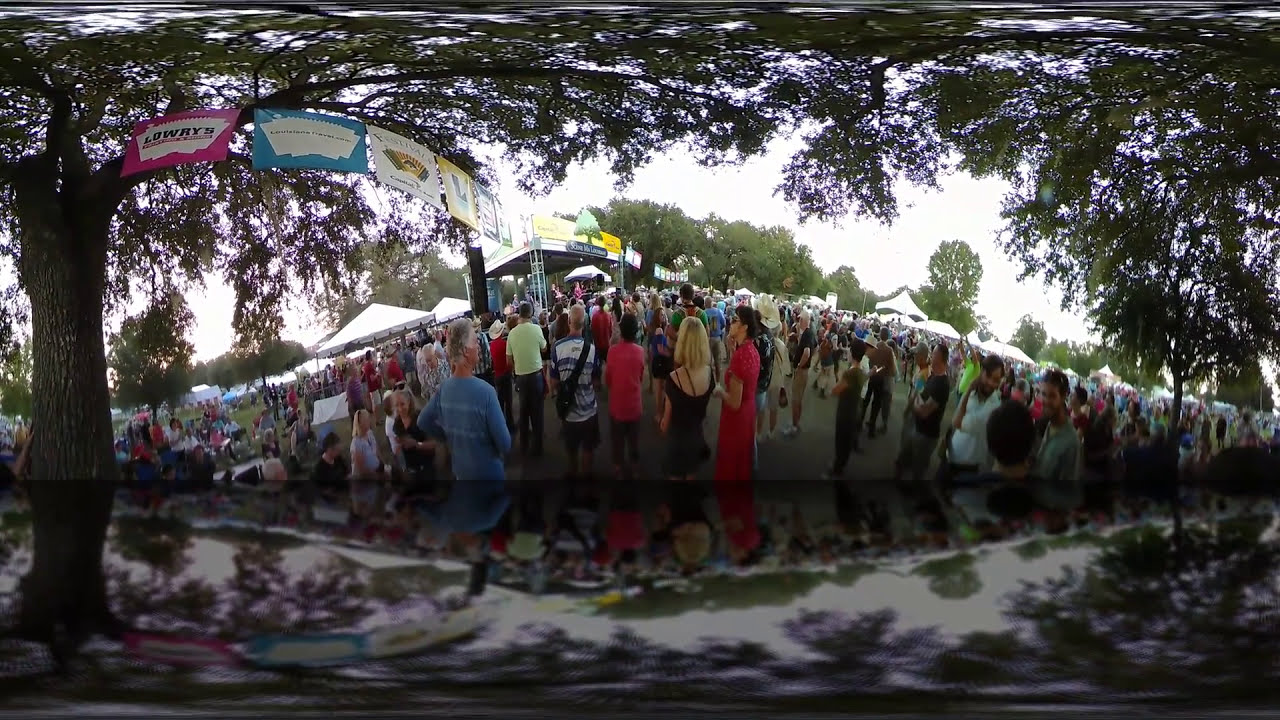The image depicts a large outdoor event, likely a festival or concert, featuring a crowd of several hundred casually dressed people. They are gathered around a noticeably warped and stretched central stage, indicative of a fisheye lens effect. The crowd is diverse, with attendees wearing everyday clothing such as T-shirts, polos, dresses, and skirts. The event is set in a park-like area with prominent greenery, including trees that appear distorted and interlaced at the top due to the lens. White tents and sheds are visible in the background, adding to the festival atmosphere. In the center stands a stage with four metal columns and a yellow roof featuring a tree design. There are several banners and signs hanging from the trees, one of which reads "Lowry's" or "Lauri's," although some text is too small to discern clearly. The festive ambience is further emphasized by people capturing memories with their cameras and phones.